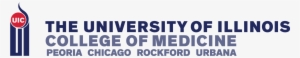The image appears to be a logo, possibly designed for inclusion on a web page or within an app, and has been cropped. It features a small rectangular background in a bluish white hue. Prominently displayed in bold, blue uppercase text is "THE UNIVERSITY OF ILLINOIS." Directly underneath, in a lighter bluish-gray uppercase font, it reads "COLLEGE OF MEDICINE." Below this, in smaller text of the same lighter bluish-gray color, the locations "Peoria, Chicago, Rockford, Urbana" are listed without conjunctions.

To the left of this text is a distinctive logo. The logo features a red circle resting on a dark blue base. Inside the red circle, there are white letters that partially spell out "U C." The dark blue base is the same hue as the "UNIVERSITY OF ILLINOIS" text. Above the base are three prongs, somewhat resembling a trident without a handle, with the rightmost prong curling upwards like a wisp of hair blown by the wind. The overall design is visually intricate and indicative of an official emblem.